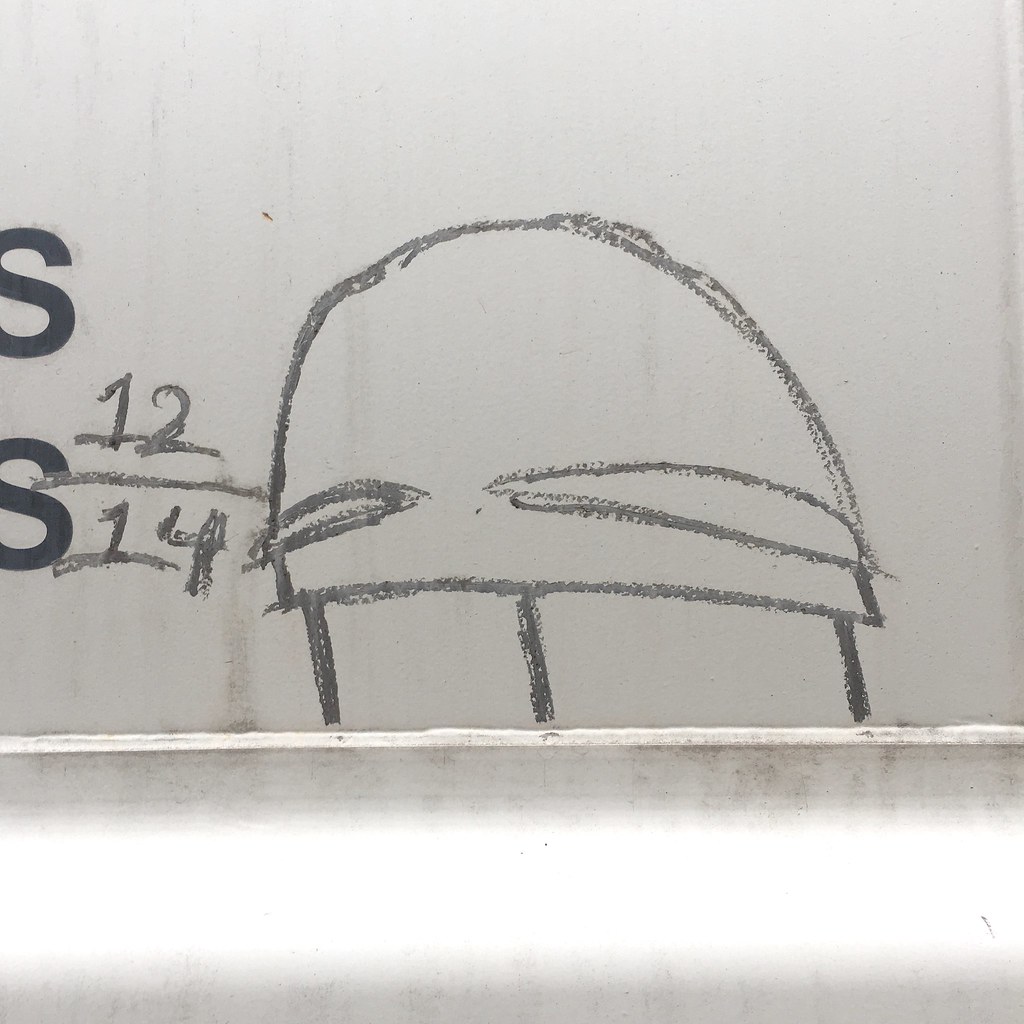This image is a slightly taller-than-wide drawing on slate gray paper, divided horizontally by a white line into two sections. The bottom section, taking up about 30% of the height, features a charcoal smear in its upper quarter, while its lower quarter remains plain white. The top section has an off-white background and contains a simple schematic drawing in gray pencil or charcoal. This drawing features a dome-like shape, slightly slanted to the left, with two long, oval shapes resembling eyes beneath it. The dome is connected to the bottom of the picture by three skinny straight lines, giving the appearance of a stem. On the left side of this drawing, "12/14" is written, and below these numbers, there are two bold uppercase black S's, one directly beneath the other.